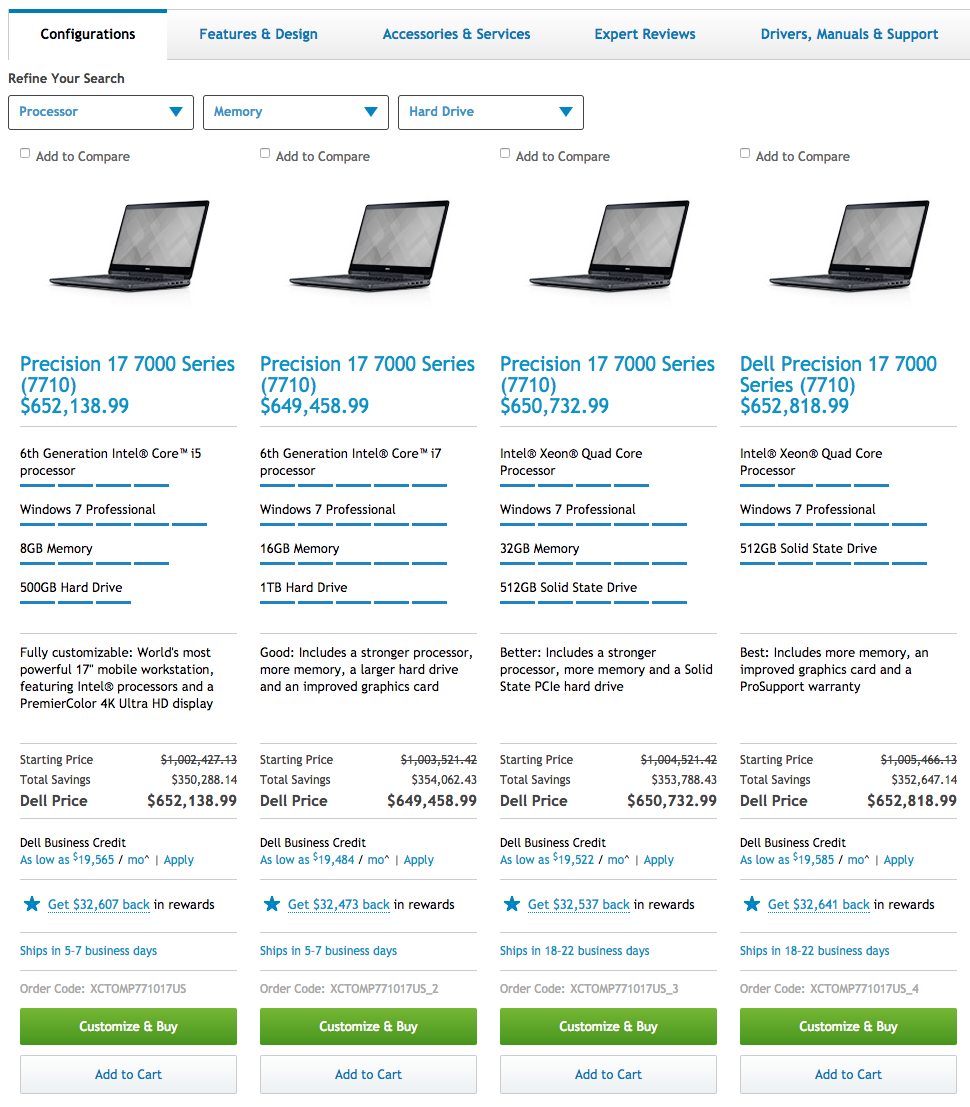This screenshot displays a Dell webpage featuring various laptop purchase options. At the top, a gray navigation bar spans across, presenting five tabs: "Configurations," "Features and Design," "Accessories and Services," "Expert Reviews," and "Driver's Manuals and Support." The "Configurations" tab is highlighted with a white background and a blue underline. Below this navigation bar are three drop-down menus, labeled "Processor," "Memory," and "Hard Drive," arranged side-by-side. Further down, four distinct laptops are showcased in four columns. Each column includes an "Add to Compare" option in the top left corner, followed by an image of the laptop and the specific model name beneath it. The highlighted model in this instance is the Dell Precision 177000 series (7710), with a striking price of $652,138.99.